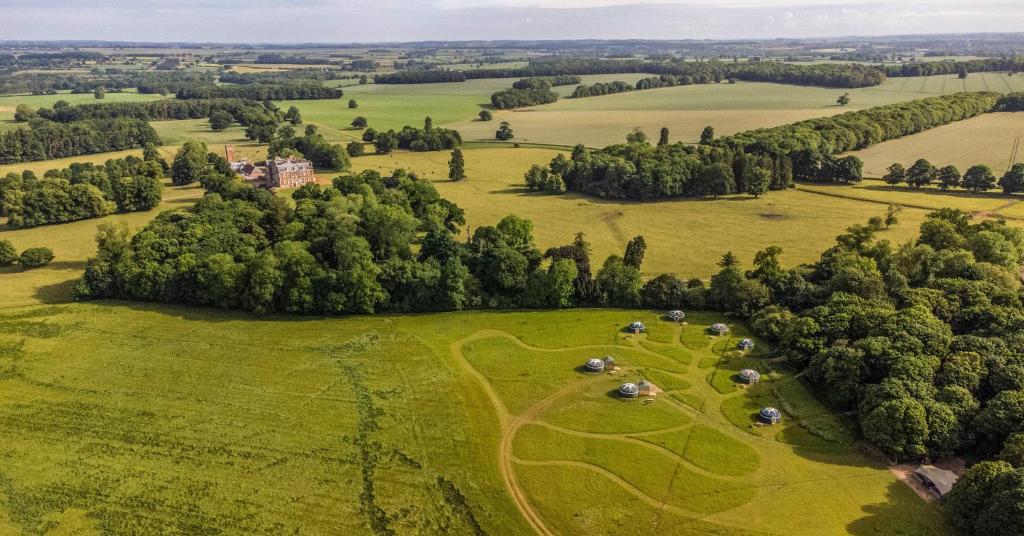This image presents an aerial view of a vast, open farmland taken from approximately 50 feet above ground. The landscape is a lush, verdant expanse of green grass, divided into several plots and pathways that weave through the fields. Prominent clusters of trees, their leaves a vivid green indicative of the height of summer, break up the landscape. Among the fields are several small structures, including a sizable house with a gray roof located towards the bottom right of the image, and multiple circular, red-brick accessory buildings scattered across the property. The horizon stretches far into the distance, just below the top of the photograph, revealing silhouettes of mountains and possibly a city or incorporated area in the far left corner. The picturesque scene is devoid of text, focusing purely on the serene natural and architectural elements.